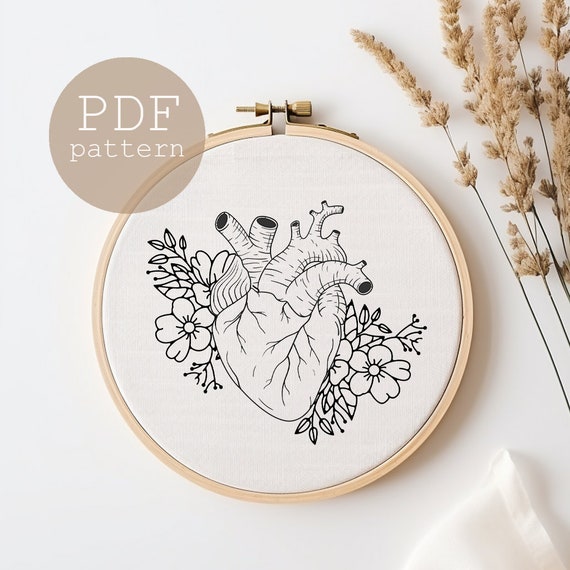This detailed close-up photo showcases an embroidery template, specifically a PDF pattern, featuring a highly detailed black and white outline of a human heart surrounded by an intricate design of flowers and leaves. The heart, depicted with visible veins and muscles, is centrally placed within a fabric circle that is stretched tightly in a wooden embroidery hoop, accentuated by a gold screw at the top. The backdrop consists of a light beige color with beige-colored wheat grains adorning the upper section of the image. The lower portion of the photo includes a white corner of cloth slightly dropping a shadow on the right side. Also present are decorative sprigs of wheat-like plants on the right, and the entire setup is resting on a white table. Additionally, a small brown circle with white text indicating "PDF pattern" is situated at the top left.